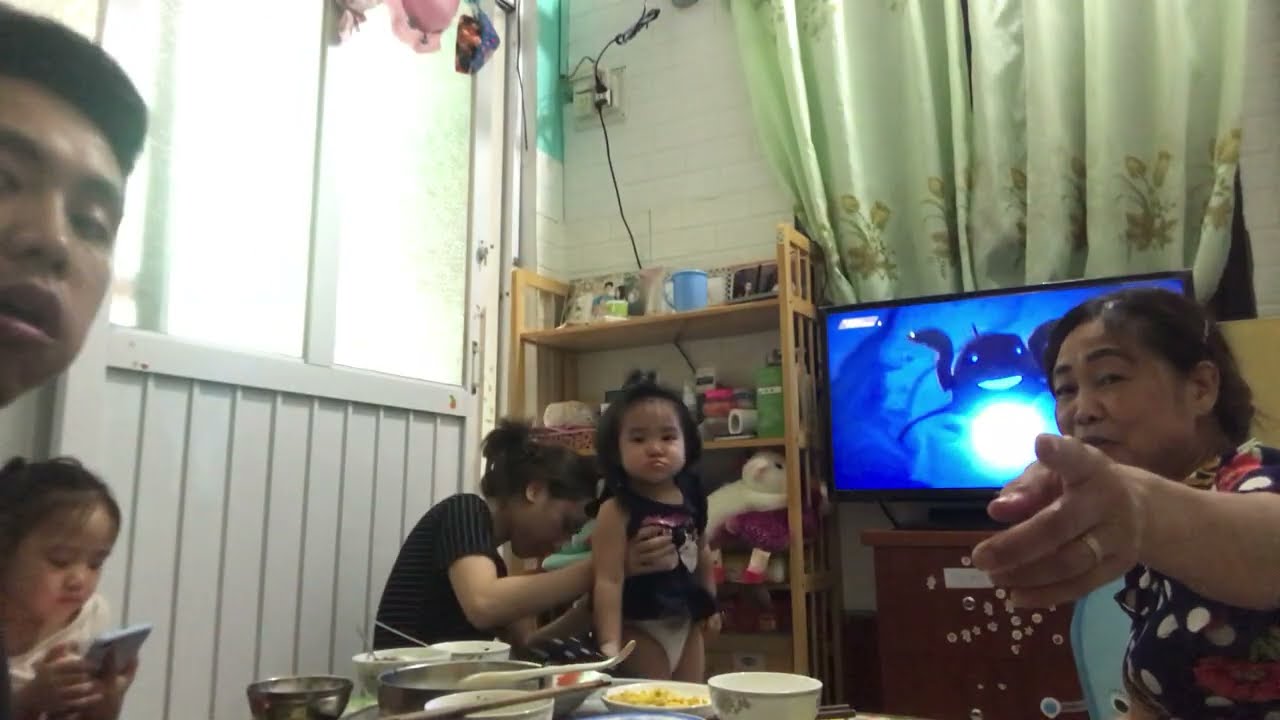This photograph depicts an intimate scene within an Asian family's home, likely of Japanese ethnicity. The room features a table at its center, laden with various food items, ceramic bowls, and metal pans, around which five individuals are gathered. The family members include an older woman, a man, two young children, and another young woman, possibly the mother.

The older woman, positioned on the right side of the image, is seated directly in front of the table. She has black hair secured with a barrette and wears a wedding band on her left ring finger. Her left arm is extended, pointing towards the camera, indicating some form of interaction with the photographer or something beyond the frame.

In the background, to the right of the older woman, there is a television displaying a cartoon, which could be "Baby Shark" or something similar. Central to the image, there is a young mother, likely in her 20s, who is fixing the outfit of a little girl around three or four years old. The mother has her hair pulled back in a ponytail or bun and is fully focused on adjusting the child's clothing, which appears to be a pink dress with black ruffles. The little girl, wearing black hair pulled back, looks directly at the camera.

On the left side of the image, partially cut off, a young man, approximately 14 or 15 years old, watches the scene and looks towards the camera. Adjacent to him, a young girl around five or six years old sits at the table, seemingly reading a book. 

The room's aesthetic includes a mix of white paneling and white brick walls, with a white-framed window above and a white door on the left side of the room. The wall also features a white silk curtain with printed flowers. A wooden shelf stands behind the family, holding various items like photographs, tissues, and towels, offering a glimpse into the personal and lived-in ambiance of the home.